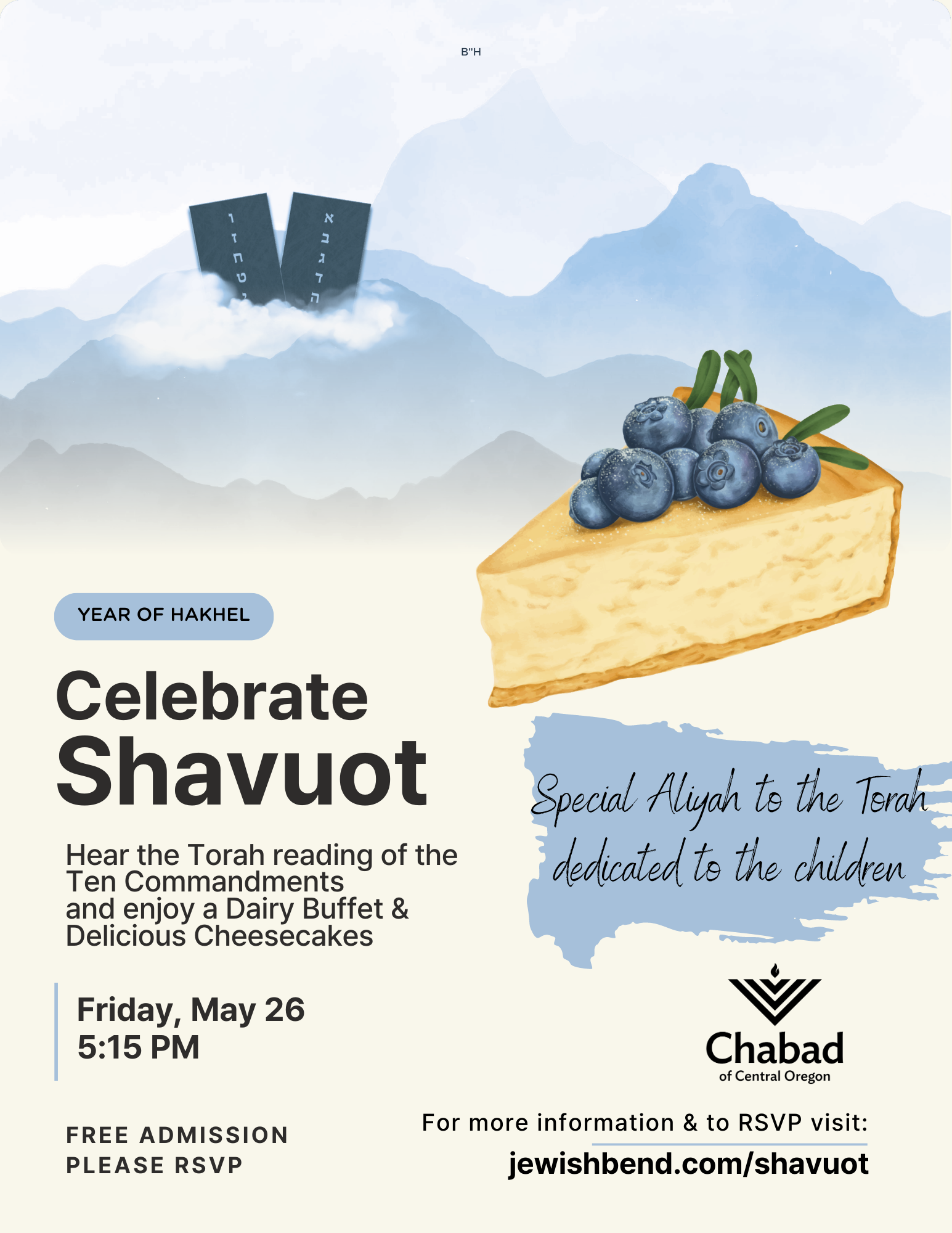The image is an event flyer for a Jewish celebration. The backdrop features a serene depiction of mountains, with layers of blue and light blue silhouettes. Clouds drift through the scene and two dark gray rectangles with text emerge from the mountain range. The centerpiece of the upper portion is a mouth-watering illustration of a cheesecake slice, adorned with fresh blueberries and green leaves, resting on a flaky crust. 

On the left side, a vertical blue band reads: "Year of Hakel. Celebrate Shavuot. Hear the Torah reading of the Ten Commandments and enjoy a dairy buffet and delicious cheesecakes. Friday, May 26th, 5:15 PM. Free admission, please RSVP." To the right, there's an artistic paint swish backdrop for the text: "Special aliyah to the Torah dedicated to the children." A logo of Chabad of Central Oregon, reminiscent of candles formed with three 'V' shapes, is also present.

At the bottom, the flyer provides further details for RSVPs and additional information, directing readers to visit jewishbend.com/Shavuot.